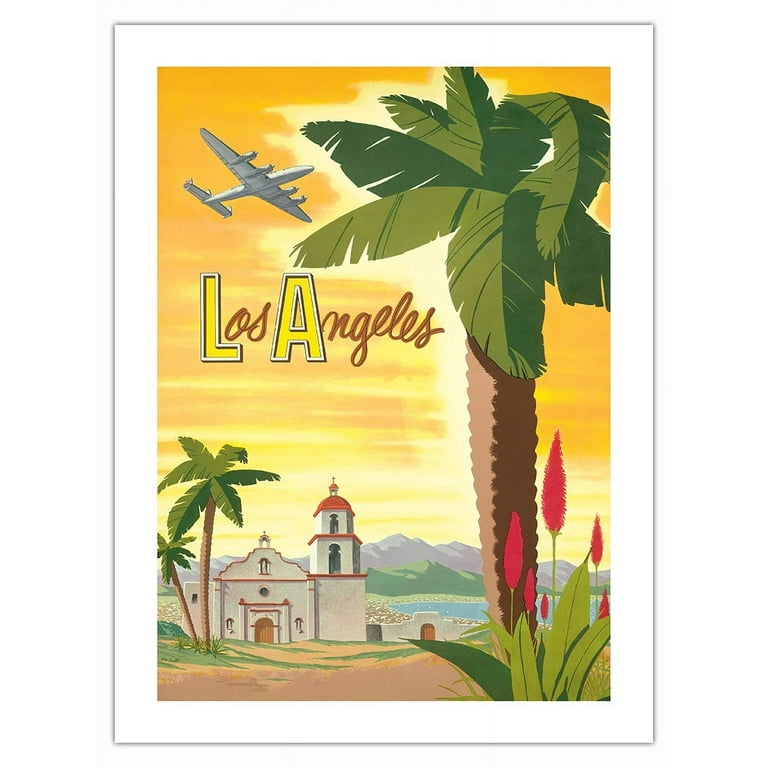This is a vintage-style illustrated poster or postcard for Los Angeles, featuring a vibrant yellow-orange sky reminiscent of a sunset. Prominently, the words "Los Angeles" are displayed across the center with the "L" and "A" in large block yellow letters bordered in white, while the rest of the text is in a smaller brown cursive script. An old-fashioned silver airplane is depicted in the upper left, flying across the sky.

Dominating the right side of the image is a large palm tree with a dark brown trunk highlighted by a lighter brown color, and fronds in two shades of green. Below the palm tree, there’s a plant with red cone-like flowers. 

To the left, a mission-style building is featured, characterized by its white walls, red-tiled roof, and mission bells. The building is flanked by additional palm trees, and in front of it, a dirt path leads toward a brown wooden gate, beyond which lies a body of water.

In the background, a series of mountains can be seen, the nearest ones green, with taller gray peaks rising behind them. A blue bay area extends to the horizon, completing the picturesque Southern California scene. White borders and dark edges frame this appealing, travel-inviting artwork.